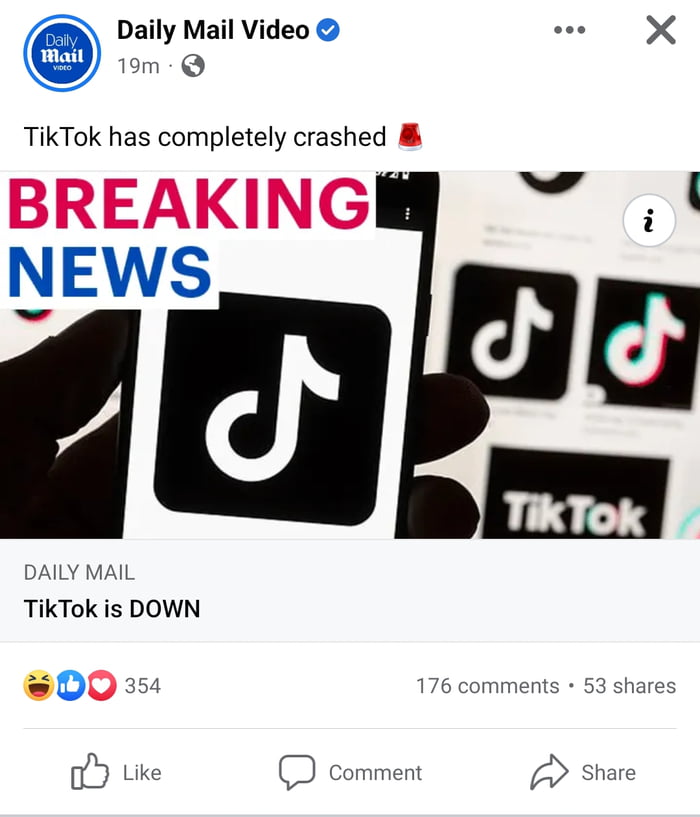A Tweet from the Daily Mail reports that TikTok has completely crashed. The accompanying image displays "Breaking News" boldly, surrounded by multiple TikTok logos. One notable graphic is a silhouette of a hand holding a phone with the TikTok app visible on the screen. The background is predominantly white, maintaining a clean and urgent aesthetic. The tweet has garnered 354 likes, 176 comments, and 53 shares in a short span of time, having been posted just 19 minutes ago. The recognizable Daily Mail logo is positioned next to the word "video," suggesting the content likely contains a video link. Additionally, there's an ‘X’ button at the top right, allowing viewers to exit and return to previous activities. A siren icon is placed near the word "crashed," emphasizing the urgency of the situation.